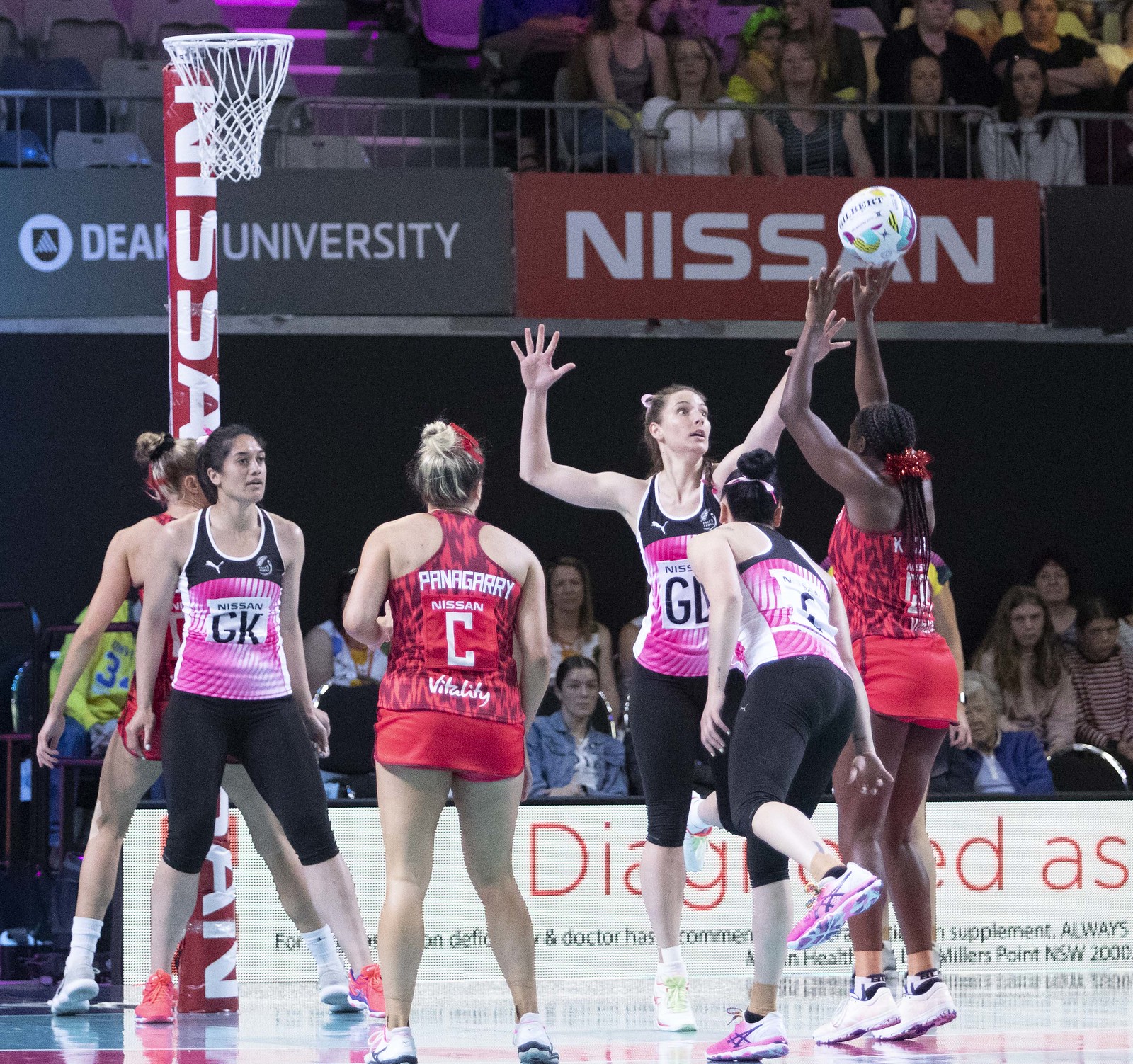This image captures an intense women's basketball game taking place in a brightly lit gymnasium with a shiny court painted in blue and red. There are six players on the court, divided into two teams: one team is clad in all-red jerseys and bottoms, while the other team wears black leggings with pink tank tops. An African American player from the red team is prominently seen shooting a white basketball with blue and red trim. The hoop, distinctly all-white, hangs on the left side of the image. Spectators fill both levels of the gym, which feature promotional signage for "Nissan" and "Dean University." Additional ads and partially visible banners are scattered in the background, adding to the vibrant atmosphere of this competitive scene.